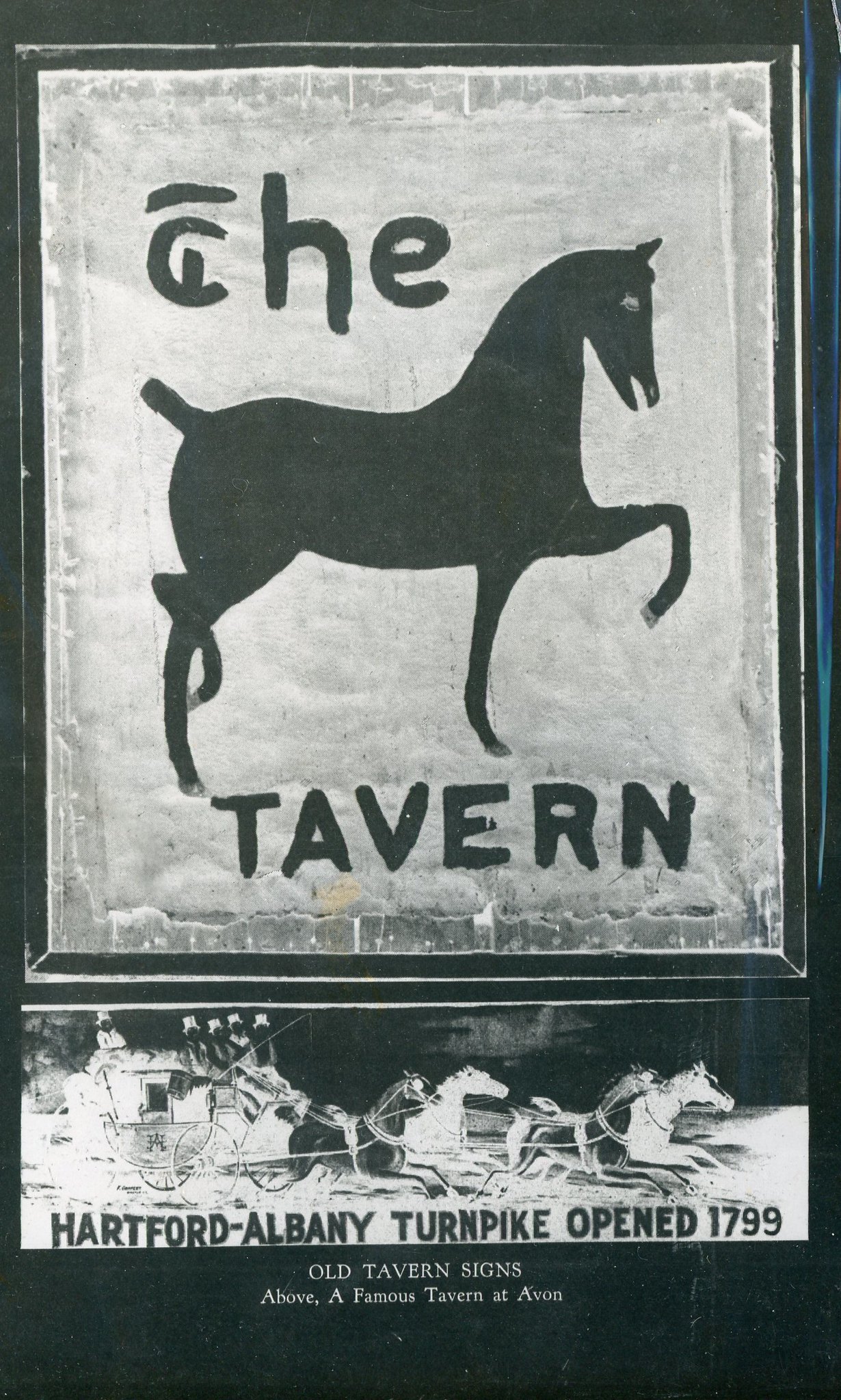The image features a historic sign for a business, prominently displaying the black hand-painted text "THE TAVERN" against a gray background. The word "THE" is positioned at the top left, with a black illustration of a horse facing right, its left hoof raised, directly beneath. Below the horse, the word "TAVERN" appears in matching black letters. The sign includes a depiction of a stagecoach pulled by four horses—black on the left side and white on the right—indicative of the transport used on the Hartford Albany Turnpike, which opened in 1799 as noted by the text below the illustration. A border frames the entire image, possibly made of metal or fabric, suggesting the sign might be a wall hanging. Additional, smaller text lies beneath the main inscriptions, though it's largely unreadable. The overall impression is that of an old tavern sign, possibly captured in a photograph, emphasizing its historic value and connection to the Hartford Albany Turnpike. The content suggests this sign might be associated with a famous tavern in Avon.